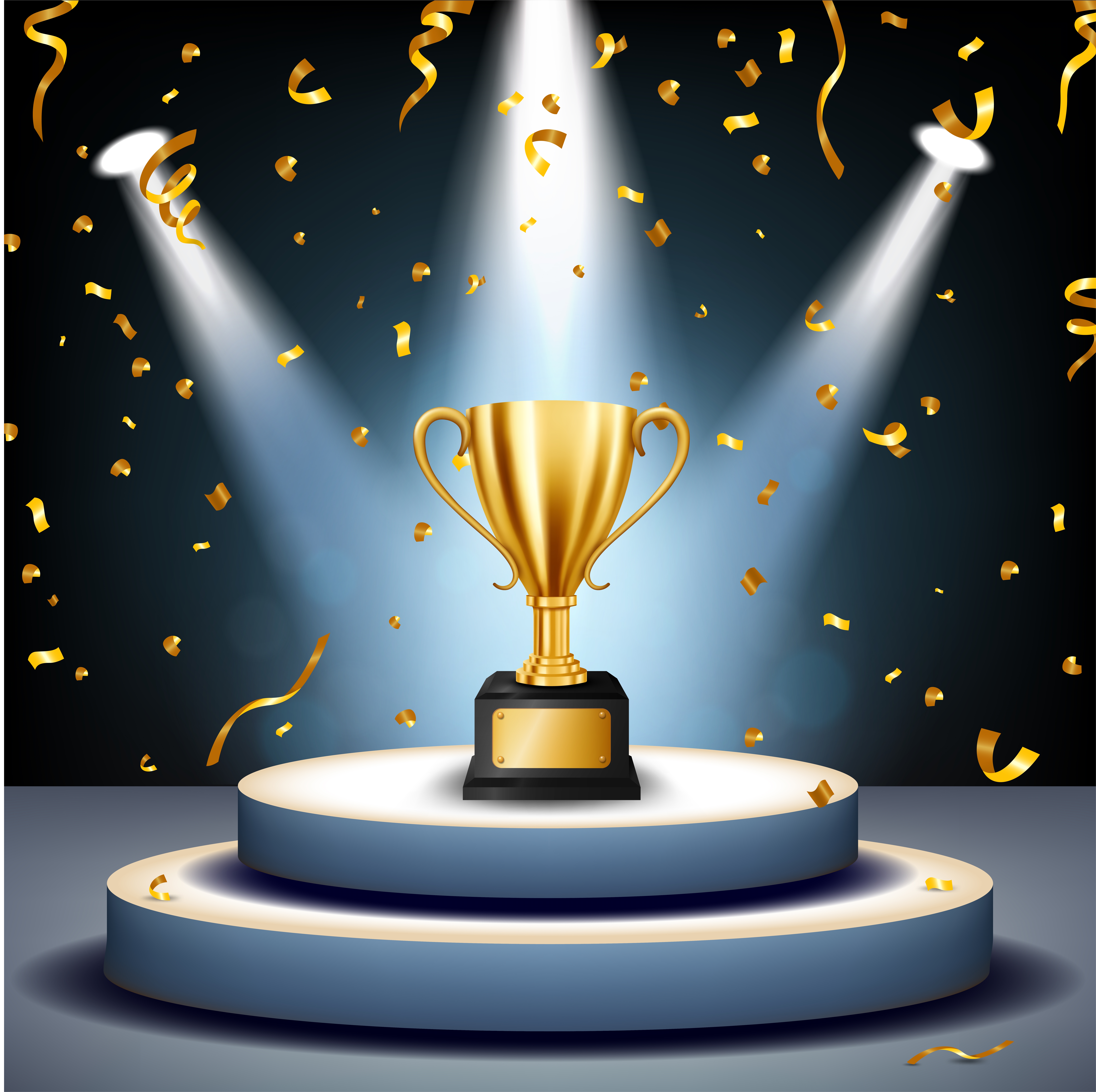The image is a digitally created, vertically rectangular scene depicting a trophy-centered composition. At the heart of the picture stands a golden cup trophy, resembling awards like the Stanley Cup, perched atop two round, white pedestals—one smaller and nested on top of a larger one—highlighted dramatically by three stage lights. The top smaller pedestal sits on the larger one, all resting on a stage or platform with gray and dark blue tones. The background features a gradient from dark blue to light blue where the lights shine, enhancing the trophy's prominence. Golden confetti rains down, some suspended mid-air and some scattered delicately on the pedestals. The setup appears as if caught in the moment of celebration, perfectly illuminated by the trio of spotlights—two angled from the sides and one directly overhead. The entire scene is clean and minimalist, with no text or additional details on the trophy's plate, evoking a sense of anticipation and high regard.